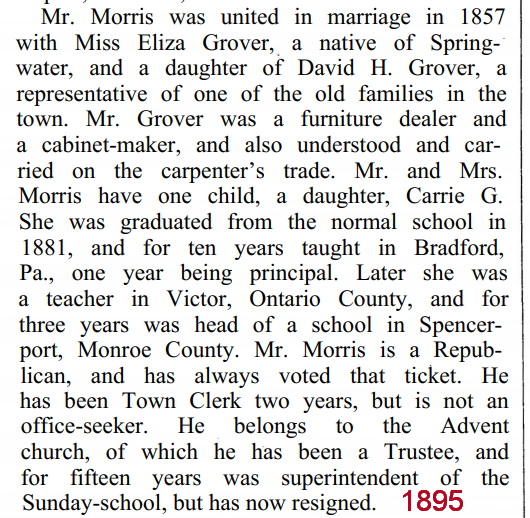The image depicts an excerpt from a book or an online article featuring a detailed account of Mr. Morris and his family. The text in black font on a predominantly white background starts a new paragraph with a slight indentation. It reads that Mr. Morris was united in marriage in 1857 with Miss Eliza Grover, a native of Springwater and daughter of David H. Grover, who was a prominent furniture dealer, cabinetmaker, and carpenter in the town. The couple has one daughter, Carrie G., who graduated from Normal School in 1881. Carrie taught in Bradford, Pennsylvania for ten years, including a year as principal, before teaching in Victor, Ontario County, and later becoming the head of a school in Spencerport, Monroe County for three years. Mr. Morris, a lifelong Republican, served as town clerk for two years and was a committed trustee and superintendent of the Sunday School at the Advent Church for 15 years before resigning.